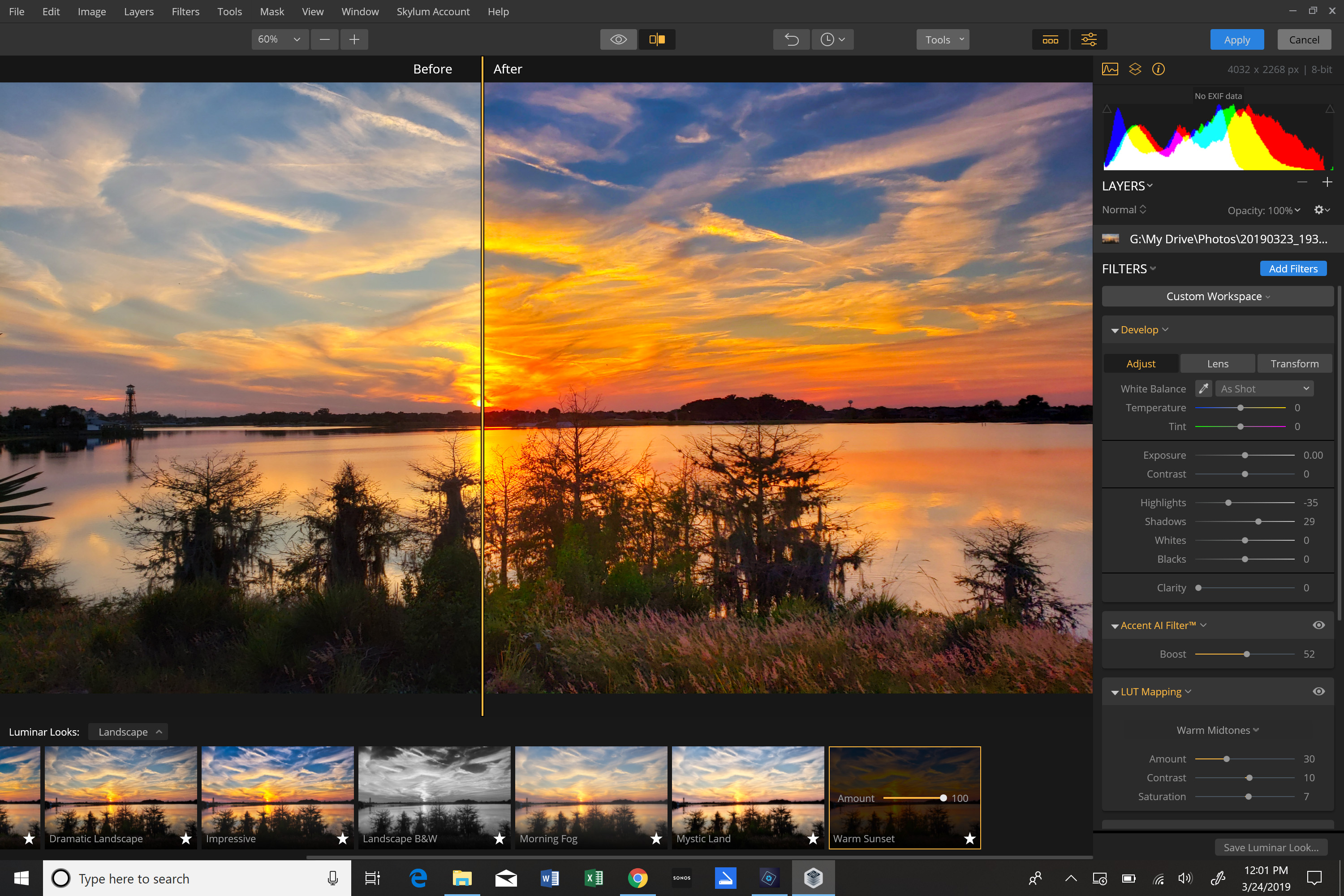A detailed screenshot captures a photo editing software interface in action. The central focus is a wide horizontal rectangular image being edited, surrounded by a dark gray workspace filled with various symbols and unreadable tiny text. The display is divided into two main sections: on the left, an outdoor scene of a lake with surrounding shrubbery and grass, supplemented by a strikingly beautiful sky. The sky starts with orange and pink hues at the horizon, transitioning into thin white cloud strips against a serene blue backdrop. The lake's water reflects the sky, adding to the tranquil ambiance of either an early morning or sunset setting.

On the right, we see the edited version of the same image. The edits have made the greenery more vibrant and detailed. Shrubs are now a richer green, and the grass appears mostly brown with some patches of green. The water reflects the vivid blue sky more sharply. The clouds have taken on deeper shades of orange, intensifying the sky’s vibrant blue.

Below these main images, a series of smaller thumbnails previewing different stages or variations of the image can be seen. To the right of the images, there is a rectangular column with an array of adjustment options. At the top, there are various color swatches and a section labeled "layers," suggesting a multi-layer editing capability. This section is equipped with sliders and dotted lines for precisely adjusting the image properties, confirming that this is indeed a photo editing interface.